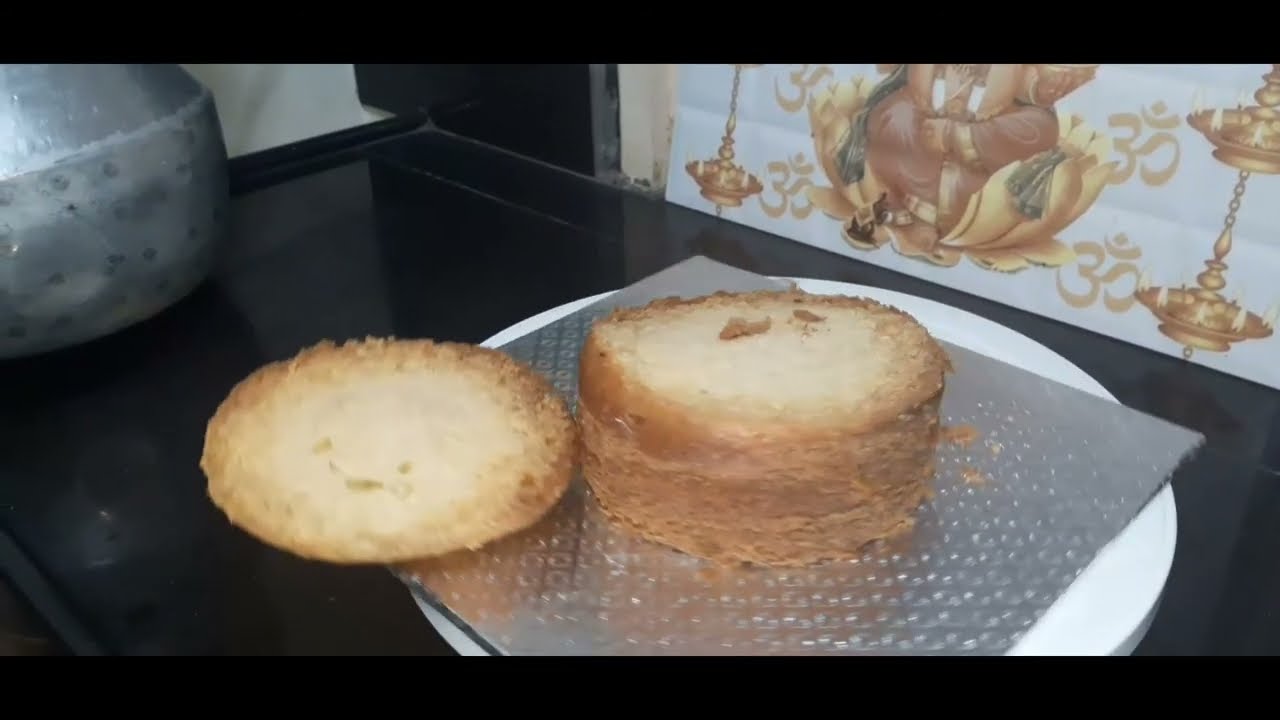The photograph captures a detailed indoor setting, possibly in a kitchen or a restaurant. At the center, there is a tan-colored, flaky cake-like pastry with its top sliced off and placed next to it. The pastry features a walled crust that is dark brown on the exterior and a lighter-colored interior. It rests on a square-shaped metallic sheet that sits on a white circular plate, all of which are positioned atop a larger rectangular black surface. To the top left, there's a partially visible shiny metal object, adding an element of interest to the scene. In the upper right corner, there is an artwork depicting a Hindu religious figure with some Hindi text, framed by what appears to be gold candelabra-like elements. The image showcases a rich palette of colors including gray, silver, black, tan, white, and green, contributing to its detailed and textured composition.